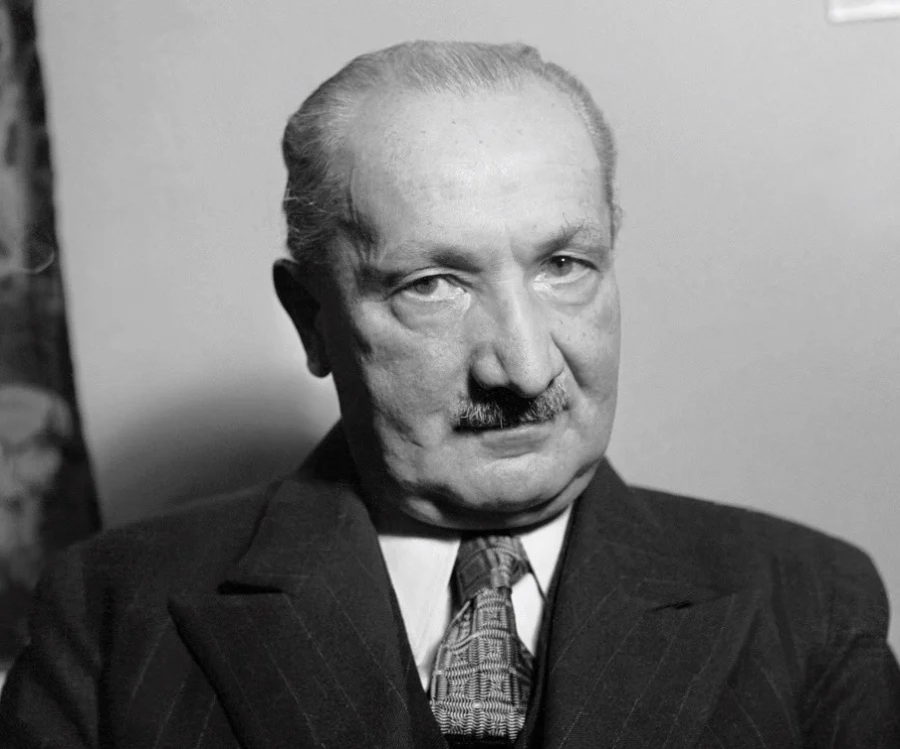This black-and-white photograph, likely taken in the 1940s, features a detailed headshot profile of the renowned German philosopher Martin Heidecker. Heidecker, appearing middle-aged, gazes directly into the camera with a stern expression that suggests he's peering into your soul. His hair, a thinning mixture of gray with hints of brown, is swept back, and he sports a medium-sized, predominantly gray mustache with a touch of salt and pepper. He is dressed in a distinguished pinstripe suit with prominently large lapels over a white dress shirt, complemented by a tie adorned with a square-like pattern. The backdrop is a simple white wall, though there is a faint, blurred presence of what might be a flag behind his right shoulder. This classic portrait captures the depth and enigmatic presence of Heidecker, offering a glimpse into his contemplative and serious demeanor.